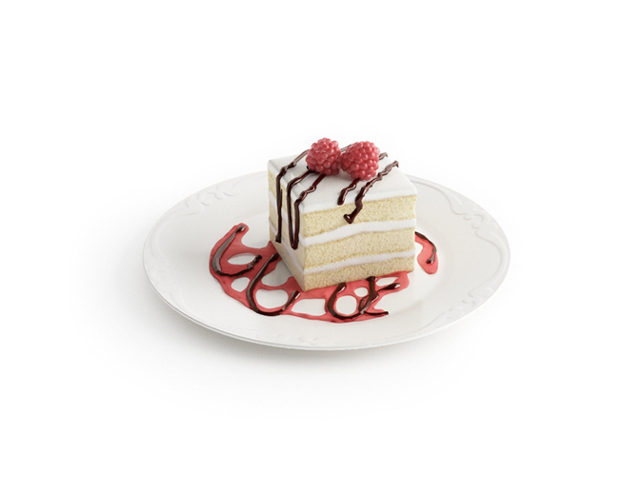This image showcases a magazine-style photo of a perfectly square piece of a three-layered white (likely vanilla-flavored) cake. Each layer is meticulously separated by a thick layer of white icing, and the cake's bread portions have a light yellowish hue. The top of the cake is elegantly decorated with a rich chocolate drizzle and two vibrant light reddish-pink raspberries. The cake sits on a small, ornate white plate, adorned with a floral scroll motif along its edge. The plate itself features additional artistic drizzles of pinkish caramel and chocolate, enhancing the presentation. The entire setup is captured against a completely white background, accentuating the cake's details and suggesting the image is intended for a cooking magazine catalog. The photograph is presented clearly, neither zoomed in nor out, allowing viewers to appreciate the full presentation.